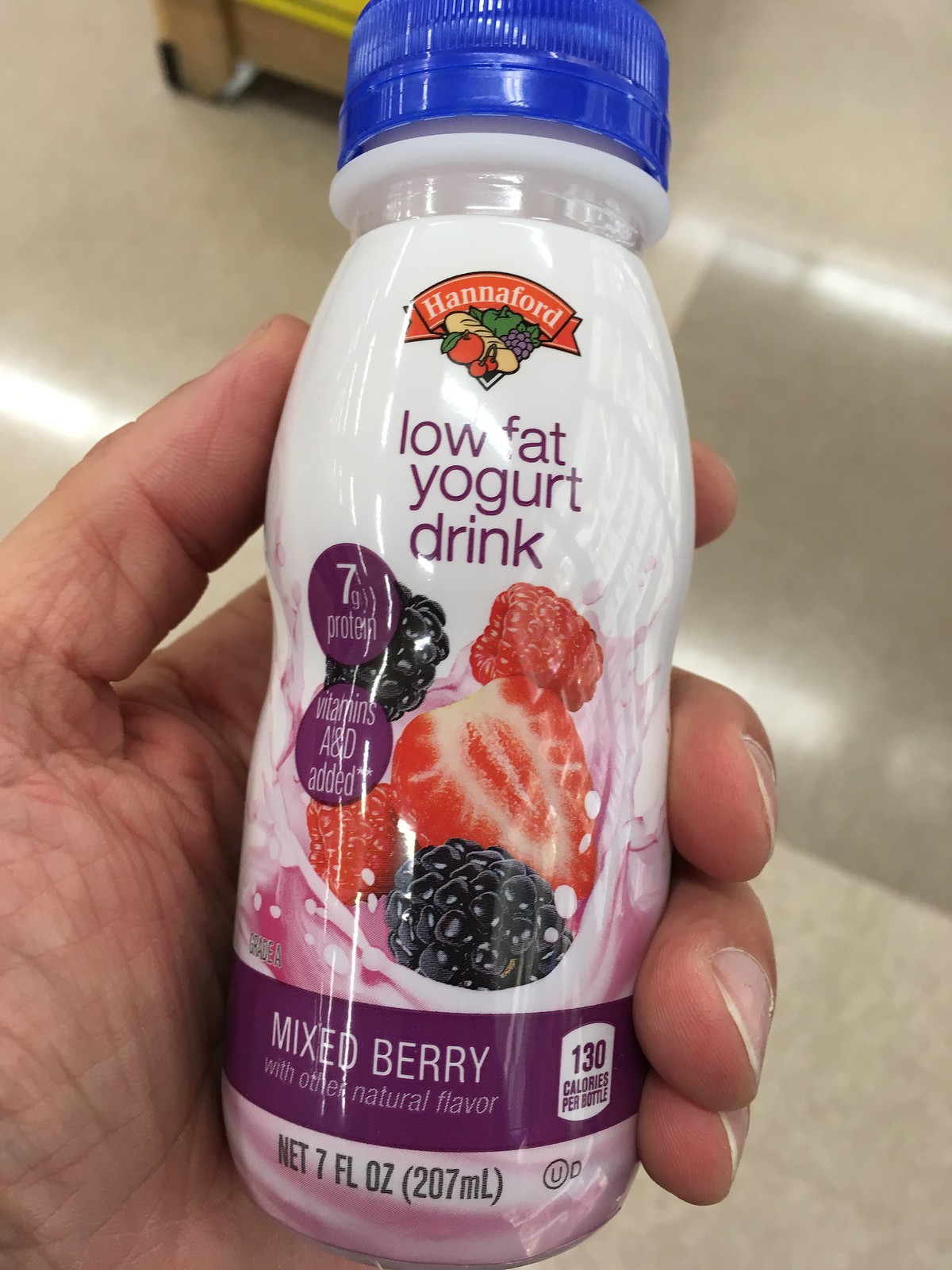A close-up image captures the masculine hand of an individual holding a small plastic drink container. The container, which is approximately the size of the hand, features a white body with a blue cap. Prominently displayed on the front is the text "low-fat yogurt drink" in a purple font. Above this, an orange banner with the brand name "Hannaford" is accompanied by colorful images of fruits, including half a strawberry, blackberries, and raspberries, depicted as if they are being dropped into a creamy liquid, emblematic of the yogurt drink.

A notable purple circle on the label highlights the product's nutritional benefits with the text "seven grams protein" in white font, while another circle indicates the addition of vitamins A and D. Below the fruit imagery, the label describes the flavor as "mixed berry with other natural flavor" and features a purple banner around the container. The dimensions of the drink are specified as "130 calories, net 7 FL OZ (207 milliliters)," providing a comprehensive overview of the yogurt beverage's contents and size.